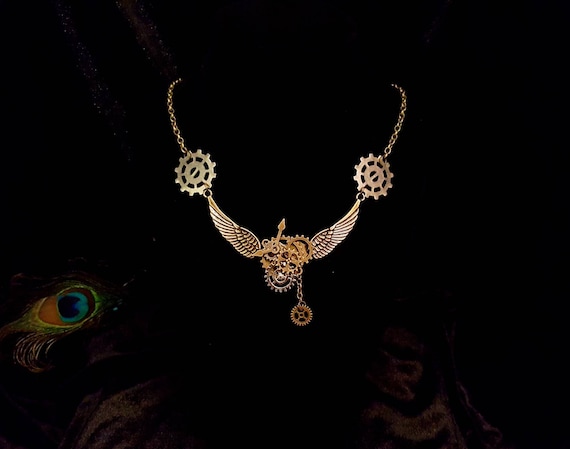The image features a striking gold necklace set against a predominantly black background. The upper part of the necklace consists of a thick, link chain. Hanging from this chain are two circular elements, reminiscent of captain's wheels or gears, with jagged, gear-like edges. In the very center of the necklace, there is an intricate pendant composed of overlapping circular gear-like pieces, further adorned with delicate angel wings extending from either side. Adding to the visual composition, the bottom left corner of the image subtly reveals a peacock feather pattern with hues of teal, blue, orange, and gold, faintly glowing against the dark backdrop. The necklace is suspended in the center, becoming the main focal point of this detailed and textured piece.